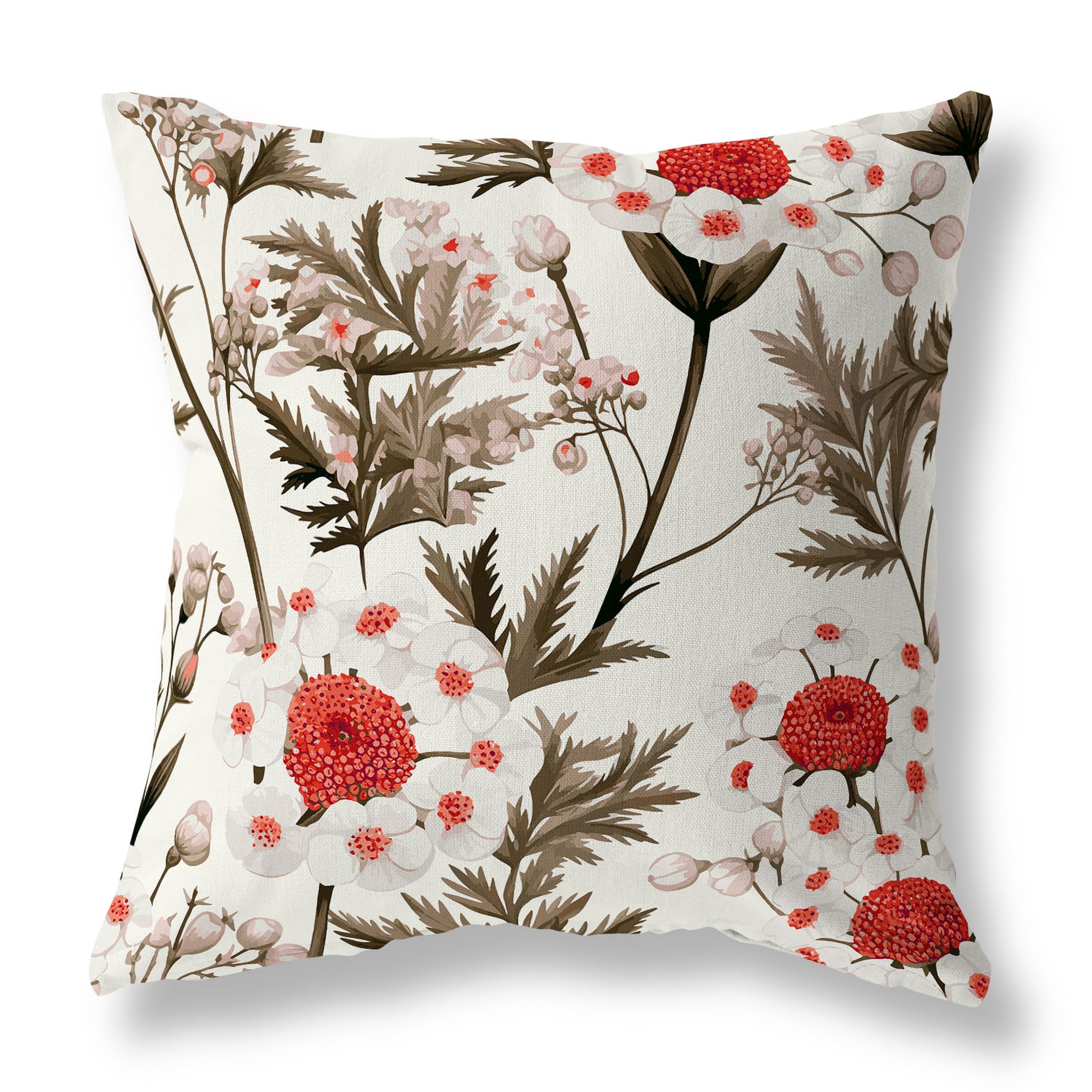This image depicts a 3D-rendered, square throw pillow that stands out against a transparent background, suggesting it is a PNG image commonly seen on product pages. The pillow boasts a distinct Japanese-inspired floral design on a white canvas. Various flowers dominate the pattern: prominent red flowers adorned with clusters of red dots and dark centers; white flowers with red centers encircling the larger blooms; and light brown flowers scattered throughout. The intricate floral arrangement is accompanied by leaves extending symmetrically from the flowers, with some green hues visible. A shadow effect along the right side and bottom of the pillow suggests light emanates from the top left, adding depth to the image. This detailed depiction highlights both the artistic and practical appeal of the pillow, making it a versatile decor piece suitable for a couch, bed, or even an outdoor seating area.